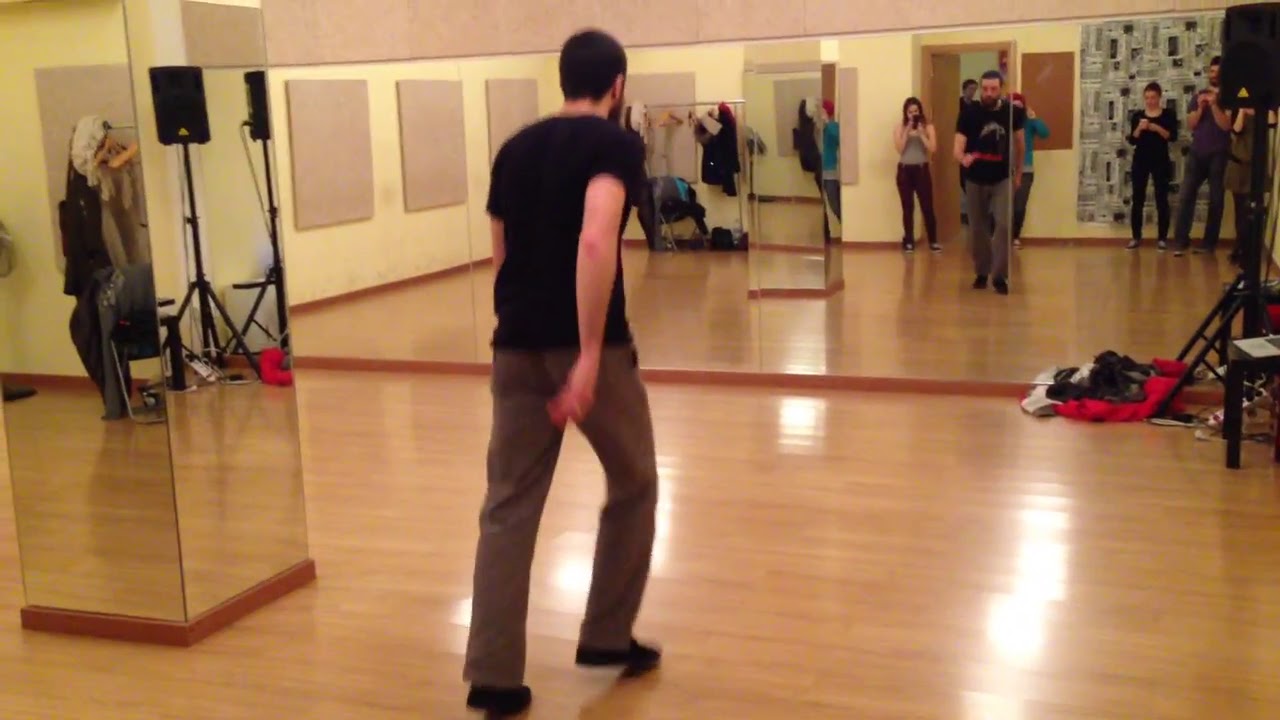In a modern dance studio or art gallery, a white man with short black hair and a beard, dressed in a black t-shirt and gray pants, steps forward towards a large wall-length mirror, his reflections capturing every move. The studio space is bustling with activity, featuring a mirrored pillar at its center and various pieces of equipment, including black speakers and clothing scattered on the floor. Approximately five onlookers, a mix of men and women, stand in the background, most holding up their phones to record or photograph the man, implying that he may be demonstrating a dance routine or leading some form of choreography. To the left of the man, a rectangular mirror-based sculpture reflects additional elements of the studio, including the speakers and more hanging clothing. Adjacent to this dynamic scene, sets of minimalistic grey paintings adorn the walls, blending the functional space with artistic elements.